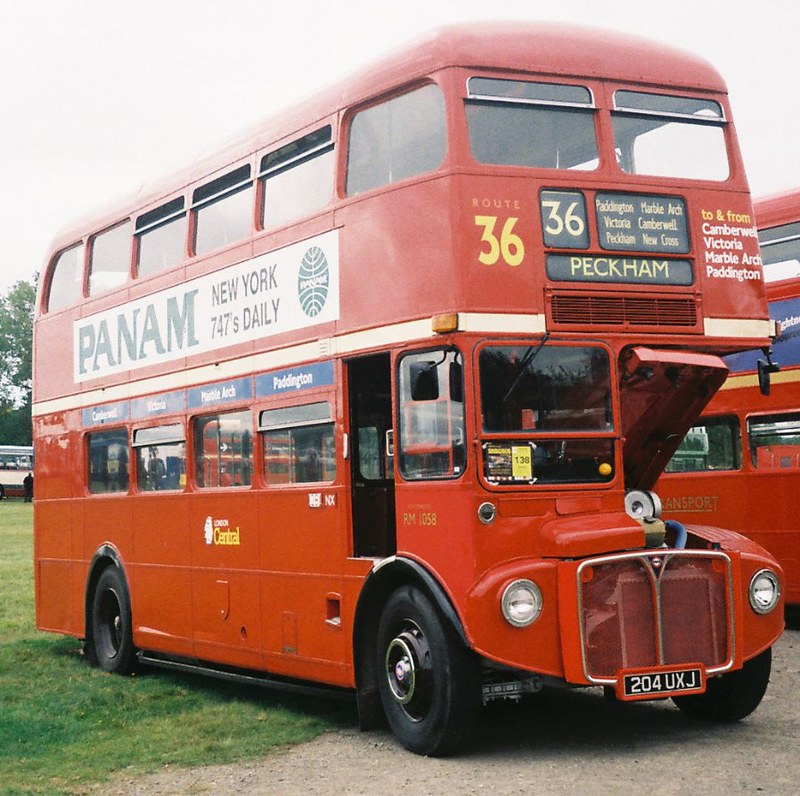In a vibrant outdoor setting, a classic red double-decker bus is parked on a road adjacent to a patch of grass. This iconic bus, characterized by its distinctive design, has a prominent black license plate bearing the registration number 204UXJ. The front of the bus prominently displays "Peckham" and "Route 36" in gold lettering on a digital display. Above this, the route details with stops such as Camberwell, Victoria, Marble Arch, Paddington, and more are listed in white on the red background, indicating its typical London route.

The right side of the upper deck features a white banner with blue lettering advertising "Pan Am New York 747s Daily," accompanied by the Pan Am logo, adding a nostalgic touch. Below the advertisement, rows of windows are visible, with the Central logo marked on the side of the bus. Another similar double-decker bus can be spotted behind it, though its details are obscured. In the background, a tree adds a touch of greenery to this quintessentially British scene. The bus appears unpopulated, with no visible passengers or driver, allowing the focus to remain on its timeless aesthetic and detailed markings.